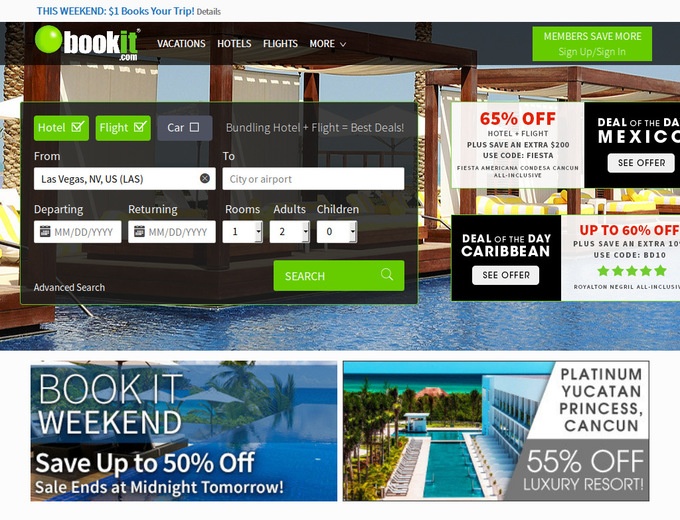This image showcases the homepage of the BookIt website. The top section features a thin light gray border, with text in blue on the top left stating, "This weekend, one dollar books, your trip," followed by a "Details" link. Below this, there is a blackish gray banner, with a green circle on the top left that includes the site’s logo "BookIt," where "Book" is in white, "It" is in green, and followed by ".com."

This section highlights various travel categories such as vacations, hotels, flights, and more. To the right, it prompts users with "Members save more, sign up or sign in."

Beneath the banner, a picturesque image of a swimming pool flanked by pergolas with white curtains flowing, creating shaded areas, is displayed. Over this image, there’s a pop-up search box with a black-gray color scheme for users to input details such as hotel and flight information, including fields for "from," "to," "departing," "returning," "rooms," "adults," and "children."

To the right of this search box, there’s a smaller box that highlights a "Deal of the Day" with a 65% discount for Mexico. Below this, another deal is advertised for the Caribbean with up to 60% off.

At the very bottom, two smaller promotional boxes are present. The left one offers "BookIt Weekend, save up to 50% off," while the right one promotes the "Platinum Yucatan Princess, Cancun," boasting a 55% discount for a luxury resort.